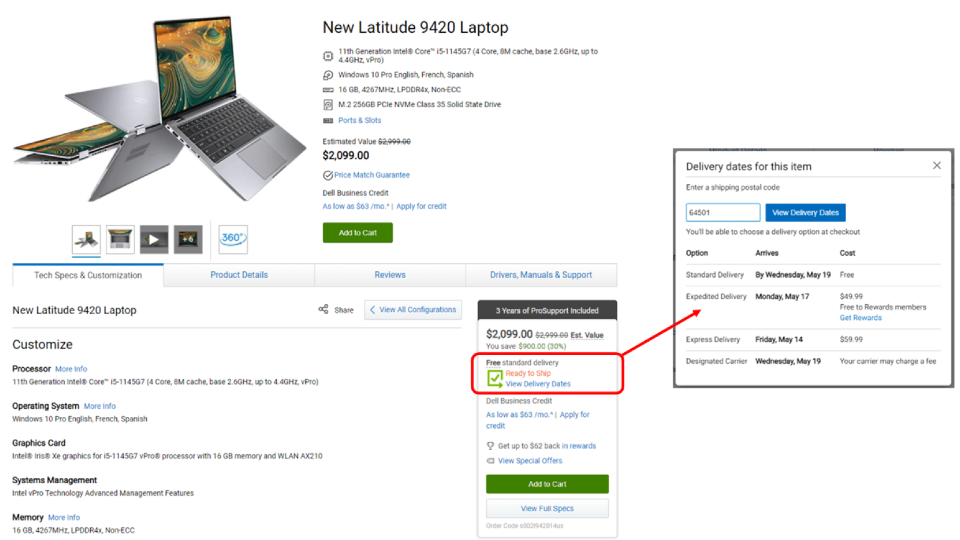This image captures a screen grab of a Dell Latitude 9420 laptop product page along with annotated details. The page is divided into two main sections: the primary webpage showcasing the specifications and price of the laptop, and an annotated section highlighting delivery options. 

In the lower left-hand corner of the webpage, within an "Add to Shopping Cart" panel, there is a red square around the "Free Standard Delivery" option. An arrow leads from this annotation to additional details about various delivery dates and costs: Standard delivery by Wednesday, May 19th is free, expedited delivery arriving by Monday, May 17th costs $49.99, and express delivery available by Friday, May 14th costs $59.99. There is also a "Designated Carrier" option for delivery on May 19th.

The Dell Latitude 9420 laptop itself is described with comprehensive technical specifications, making this screen grab a detailed focal point for potential buyers seeking both product and shipping information.